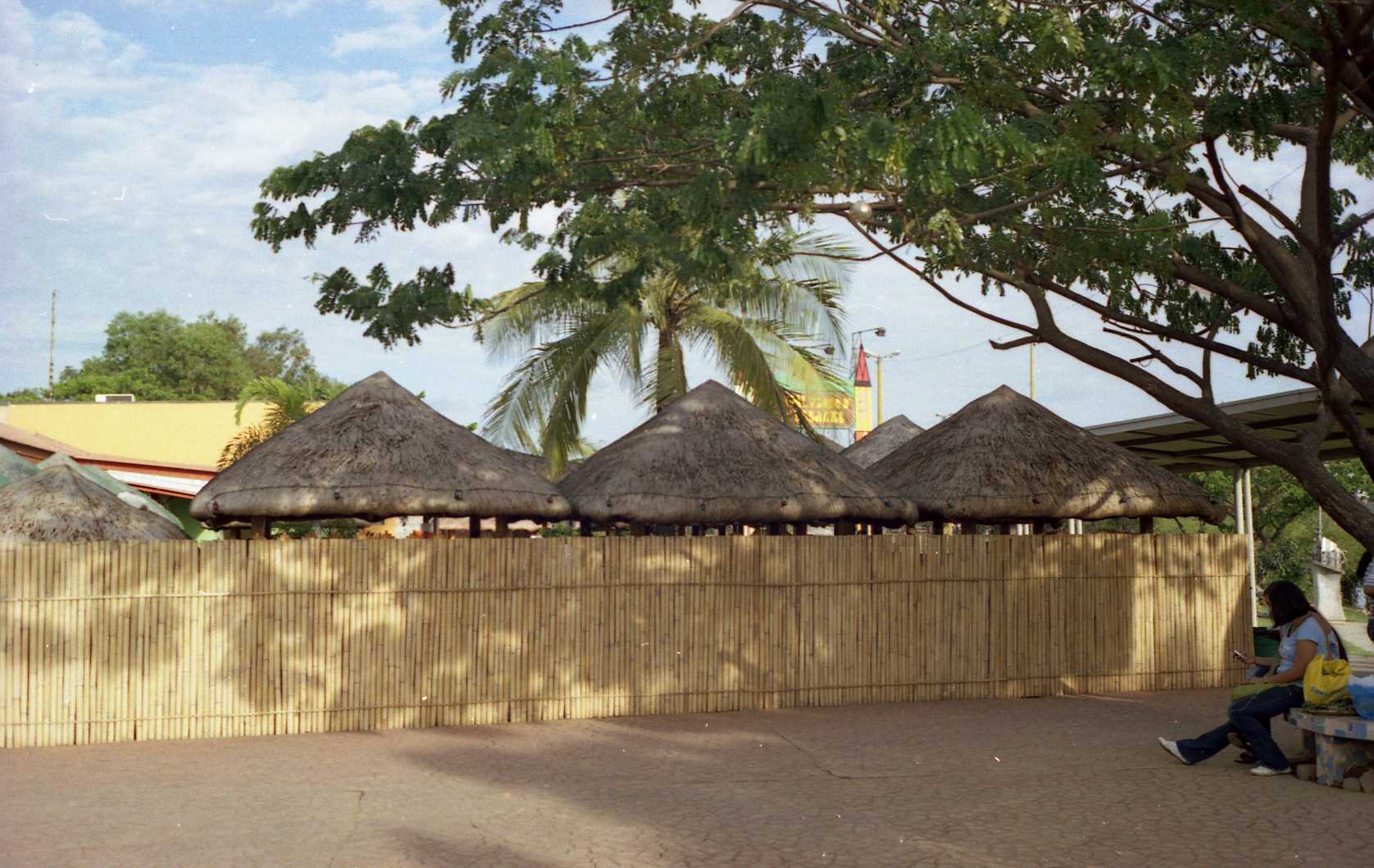In this image, we observe a sunlit, open area that exudes a tropical vibe, highlighted by the prominent palm tree in the background. Central to the scene is a wooden gated fence, marking the main focal point. Behind the fence, a collection of small huts or teepee-like structures is visible, their roofs peeking out above the barrier. This setting, likely in a foreign country distinct from the United States, features a bright day with a blue sky scattered with clouds. 

In the foreground, a tree stretches from the right center to the top center and right corner of the image, adding depth and framing the view. On the lower right side, a young woman sits on what appears to be a concrete bench, possibly engaged with a cell phone. Next to her, another individual can be seen, also seated, which reinforces the public nature of the area. The overall scene captures the serene and communal atmosphere of this tropical, sun-drenched locale.